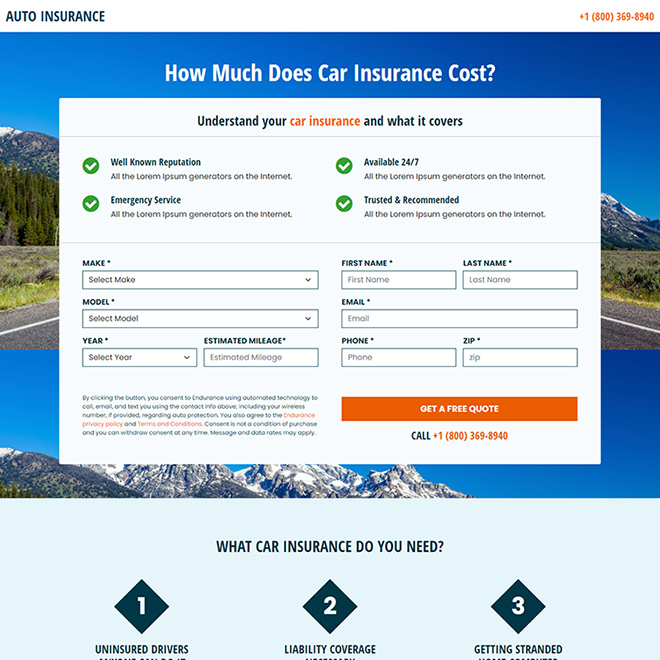The webpage is a screenshot from a car insurance comparison site. Dominating the upper half of the page is a large rectangular box with a scenic photo background, possibly depicting a road with mountains or water on each side. Overlapping this background is a white text box divided into two columns. The left column contains fields for entering car-related details such as make, model, year, and estimated mileage. The right column is designed to collect personal information: first name, last name, email, phone number, and zip code. At the bottom of the right column, there is an orange button with white text that says "Get a Free Quote."

The top of the page features a white banner against a blue sky background with the question, "How much does car insurance cost?" Below this, a darker blue header reads "Understand your" highlighted by orange text "car insurance," followed by "and what it covers" in dark blue. 

Within the white section containing text boxes, small green circles with white checkmarks indicate "Available 24-7" and "Trusted and recommended." 

Towards the bottom of the page, a pale blue section spans the width of the site, titled "What car insurance do you need?" Three numbered black diamond icons with white numbers represent different types of coverage: one for uninsured drivers, two for liability coverage, and three for getting stranded. This detailed layout aims to help users easily navigate through obtaining a car insurance quote.